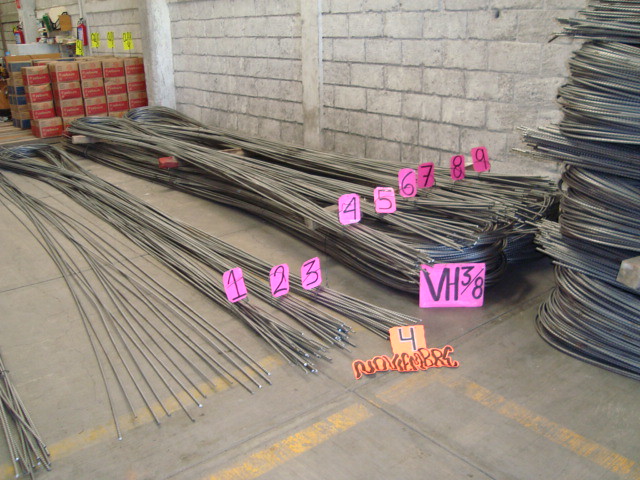The image depicts the interior of a concrete building, likely a construction site or warehouse. The white cement block walls frame the space, which is illuminated brightly by natural light. On the floor, bunches of steel rods are organized in heaps and individually arranged with pink paper labels displaying numbers from 1 to 9. Some rods also have specific markings such as "VH3-8" and the word "NOVEMBRE" written in yellow alongside the number 4. The floor is gray concrete with yellow striping, adding to the industrial feel of the setting. Additionally, there is a presence of coiled metal cables, adding variety to the materials scattered across the floor. In the background, multiple cardboard boxes are neatly stacked, further emphasizing the organized yet busy nature of this indoor workspace. The overall color palette includes shades of silver, gray, red, brown, yellow, pink, and blue, contributing to a vivid and detailed scene.